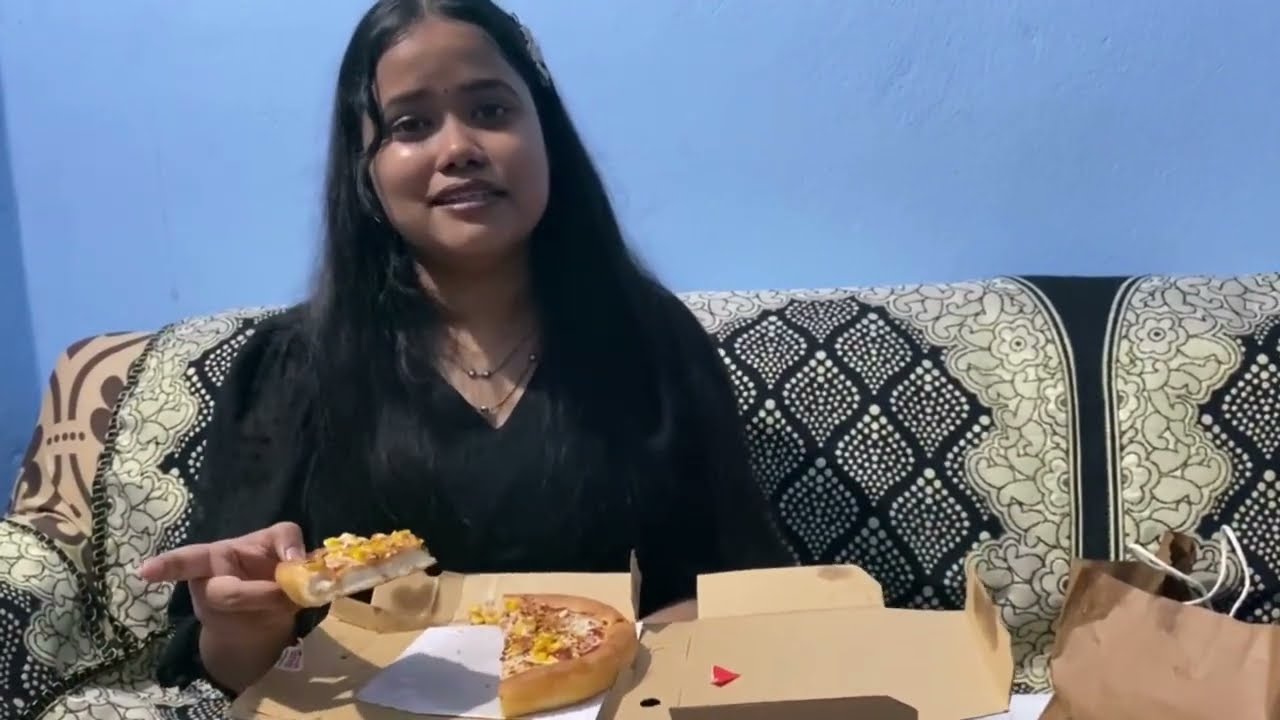The image features a woman with long blonde hair, wearing a black shirt, as she eats a piece of deep-dish pizza. She is seated on a brown couch adorned with various patterned blankets and armrest covers, set against a blue wall. In front of her is an open pizza box, revealing a small, personal-sized deep-dish pizza with half of it already eaten. The woman is looking directly at the camera while holding the pizza in her left hand and pointing to something off to her right. To her left, on the right side of the image, a brown paper bag with two white handles, presumably used to carry the pizza, rests next to her. The scene suggests a casual, homey atmosphere, possibly capturing a mukbang or a relaxed dining moment.